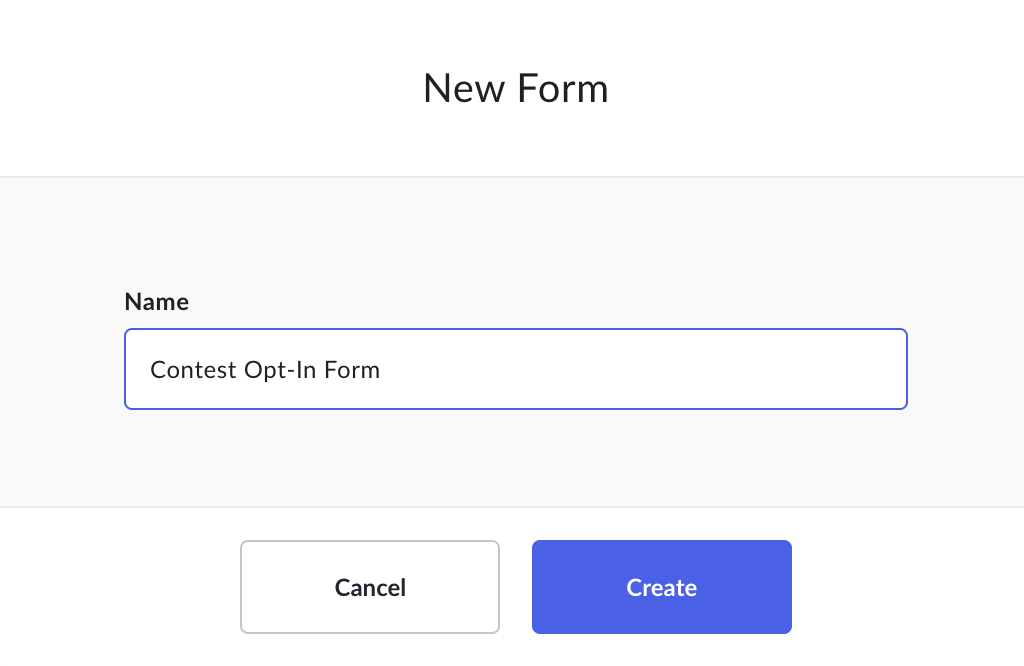This image appears to be a screenshot taken on a computer or smartphone. At the top is a white header section, prominently displaying the text "New Form" in black. Directly below this, there is a large gray rectangle that spans the width of the image. Positioned in the center of this rectangle is a white input bar with a distinct blue outline. Above this bar, in the upper left corner, is the label "Name." The input bar itself contains the text "Contest Opt-In Form."

Beneath this gray rectangle, the image continues with a white background. At the bottom of the rectangle are two buttons spaced slightly apart. The button on the left is outlined in gray, has a white background, and features the text "Cancel" in black. The button to the right is blue with white lettering, displaying the word "Create." These buttons are clearly defined and are separated by a small amount of white space.